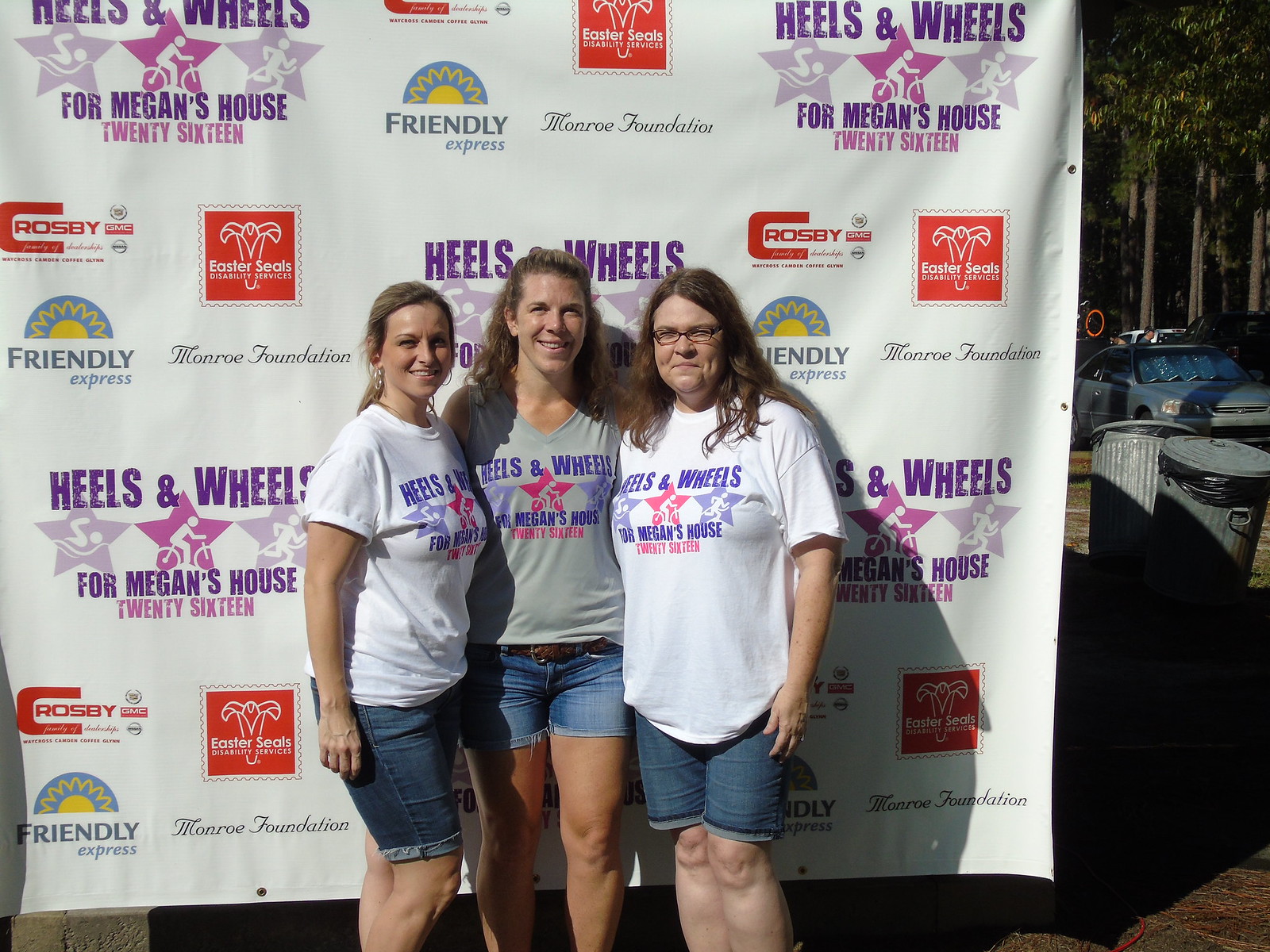Three young women stand outside in a parking lot, posing in front of a large white fabric banner covered in various sponsor logos. The banner prominently displays the event's name, "Heels and Wheels for Megan's House 2016," in purple lettering, with smaller logos for brands like Friendly Express, Monroe Foundation, Easter Seals, and Crosby GMCO repeated throughout. The women are all dressed in matching white t-shirts with "Heels and Wheels" written on them, followed by a design featuring two blue stars and one red star. Although the text under the stars is too small to decipher, the matching outfits and backdrop clearly indicate their participation in the same event. Each woman wears blue jean shorts, and they all have light brown, somewhat curly hair; the one on the left sports a ponytail, and the one on the right wears glasses and earrings. In the background, to the right edge of the image, a gray four-door car with a sun visor can be seen, along with two old-style trash bins and a row of green trees in the distance. The ground appears to be a dark brown wooden floor, visible at the bottom right corner of the image. The overall atmosphere suggests a casual outdoor event on a bright day.